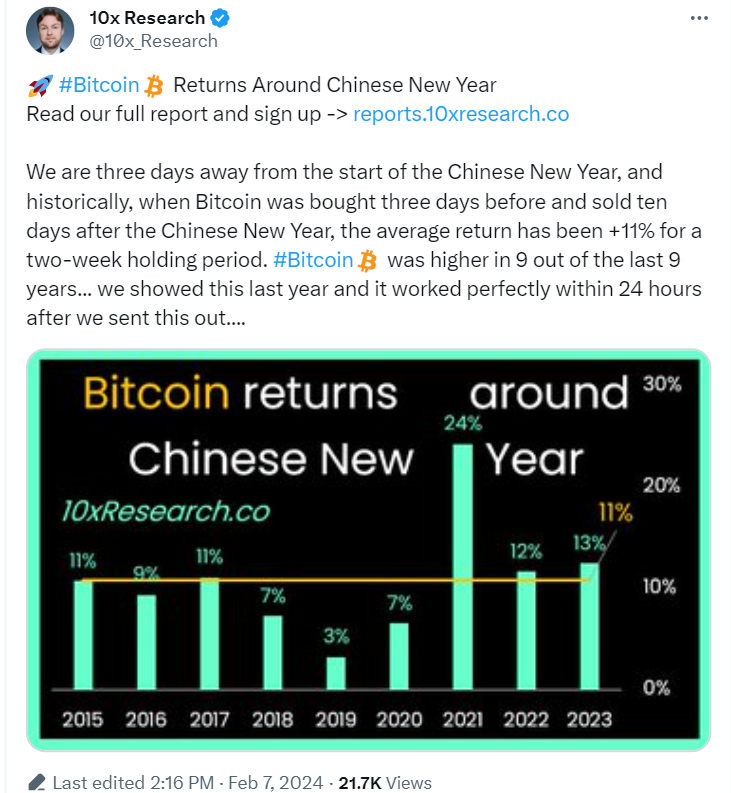This image is a screenshot of a webpage created by "Ten Times Research," verified by a blue circle with a check mark. The page features an icon of a Caucasian man with a beard and possibly a thin mustache, dressed in a suit with a button-down white shirt.

The main content of the webpage includes a detailed report titled "Bitcoin Returns Around Chinese New Year." Below the title, there is a hashtag, #BitcoinReturns, and a prompt to read the full report and sign up at reports.tentimesresearch.co.

The report highlights a significant finding: Historically, Bitcoin bought three days before and sold ten days after the start of the Chinese New Year yields an average return of 11% for a two-week holding period. The data reveals that Bitcoin had positive returns in nine out of the last nine years, with a notable increase of 24% in 2021. This pattern has been consistent from 2015 to 2023.

Accompanying the text is a large black box outlined in light green, featuring a green bar graph illustrating Bitcoin's performance over the specified years. The image was last edited at 2:16 PM on February 7, 2024.

This comprehensive analysis underscores the potential profitability of trading Bitcoin around the Chinese New Year, based on historical market behavior detected by "Ten Times Research."